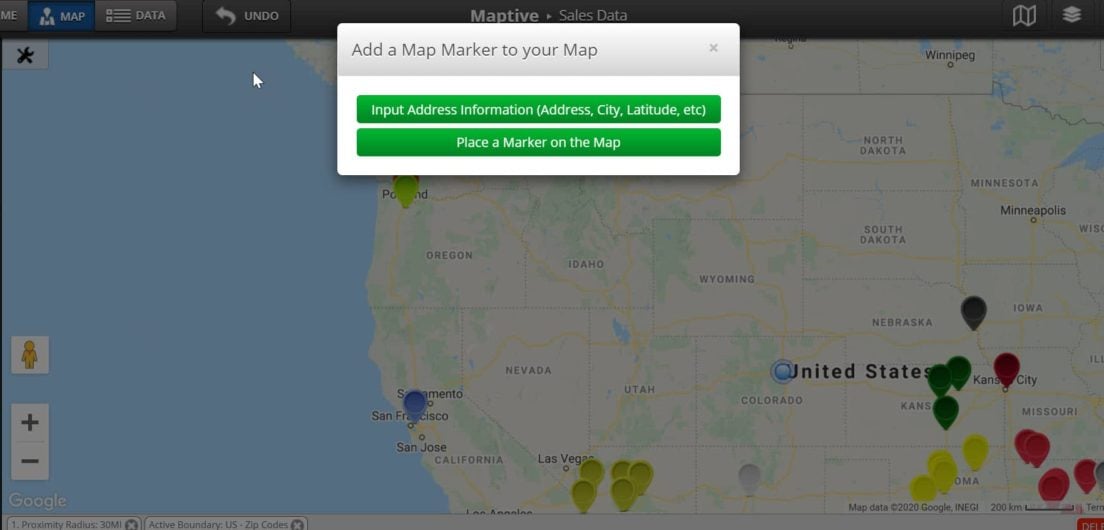A screen capture displaying an older version of a mapping program, likely Maptive. The background features a map of the central to western United States, dotted with various colored markers—purple, red, yellow, and light green—concentrated along the west coast and central plain states. The map includes faint controls on the left side for adjusting magnification. Overlaying the map is a prominent pop-up window occupying the upper half of the image. The window, which is a white rectangular box with green buttons, displays the text "Add a map marker on your map." Below this, it provides input fields for address information such as address, city, and latitude. Another green button labeled "Place marker on the map" is present. The header in the background contains the text "MAPTIVE," indicating the map software. The overall appearance suggests that this is an older interface, characterized by its dated graphical style and design elements.